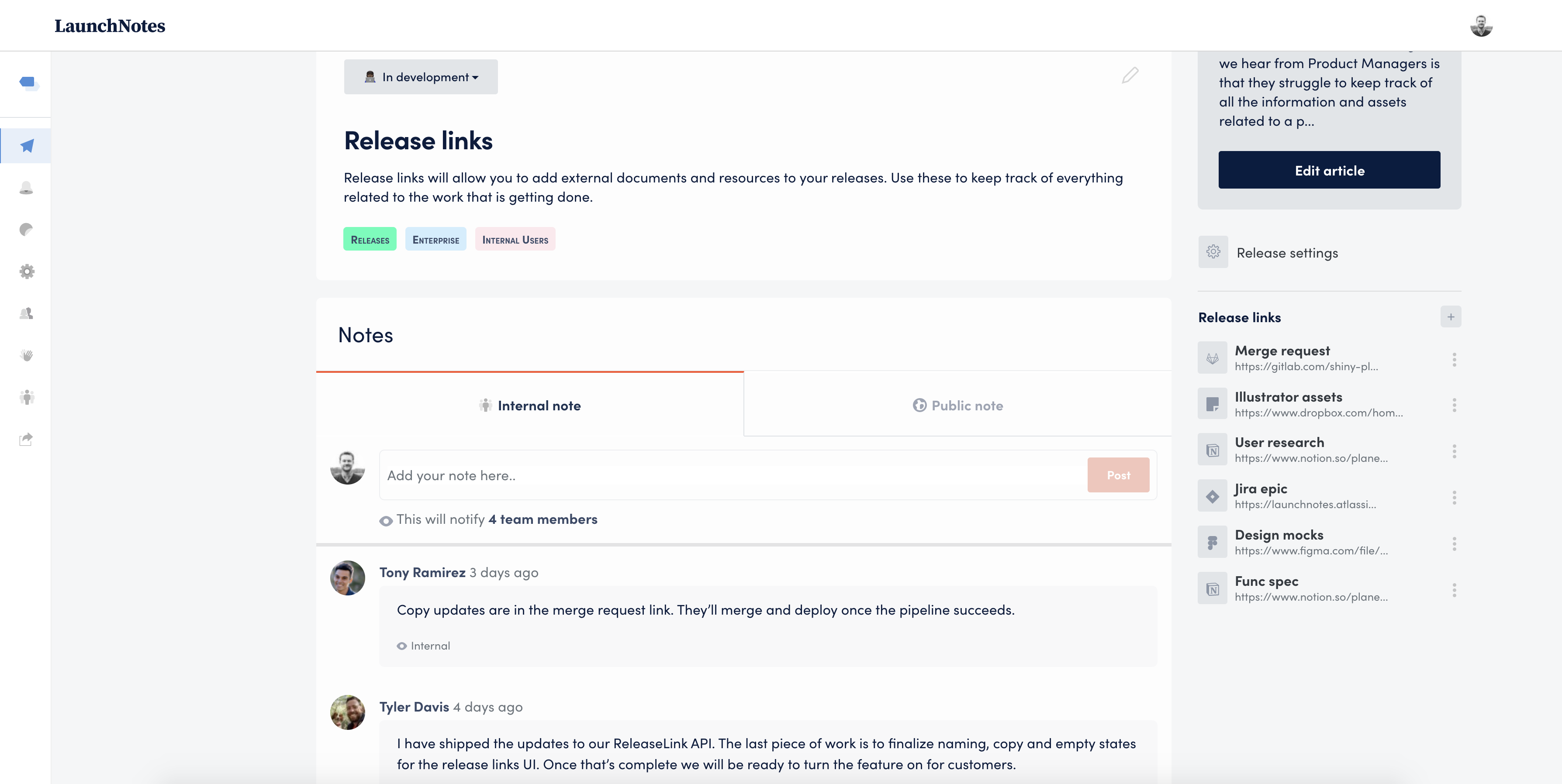Screenshot of Launch Notes Section

The image depicts a screenshot of a notes section titled "Launch Notes" located at the top left of the screen. In the center, starting from the top, there's a gray box labeled "In Development." Below this, the header "Release Links" is prominently featured, accompanied by a detailed description: "Release links will allow you to add external documents and resources to your releases. Use these to keep track of everything related to the work that is getting done."

Further down, the section labeled "Notes" appears. Here, a subsection titled "Internal Note" contains a text box with the placeholder text "Add your note here," indicating that adding a note will notify 14 members. The caption continues with an entry attributed to Tony Ramirez, dated three days ago, stating: "Copy updates are in the merge request link. They'll merge and deploy once the pipeline succeeds."